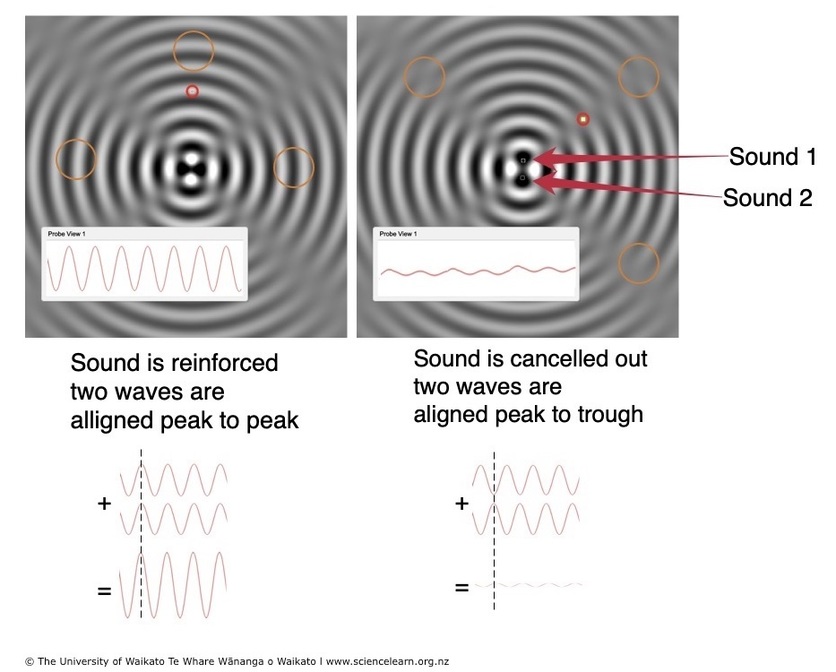This image is a scientific diagram from the University of Waikato, illustrating the behavior of sound waves using two side-by-side black-and-white pictures. Both images feature concentric circles that resemble ripples created by a pebble dropped into water. The circles start small at the center and grow larger outward, with additional little red circles with yellow spots scattered within, and some yellow circles around them too. 

The left image is labeled "Probe View 1" and depicts sound waves with high peaks and valleys, suggesting strong wave activity. Below, in black text, it says "Sound is Reinforced. Two waves are aligned peak to peak." This indicates a scenario where the waves' peaks and troughs match, amplifying the sound.

The right image also has concentric circles but with much shallower peaks and valleys, as indicated by the more consistent, squiggly red line across it, labeled "Sound is Cancelled Out. Two waves are aligned peak to trough." This demonstrates a scenario where wave peaks align with troughs, canceling each other out and diminishing the sound. 

Additionally, there are red arrows pointing towards the center of the right image, with labels "Sound 1" and "Sound 2," and both images include a white box with charts illustrating the wave patterns.

At the very bottom, the image is credited to the University of Waikato (www.sciencelearn.org.nz), marked by a copyright symbol.